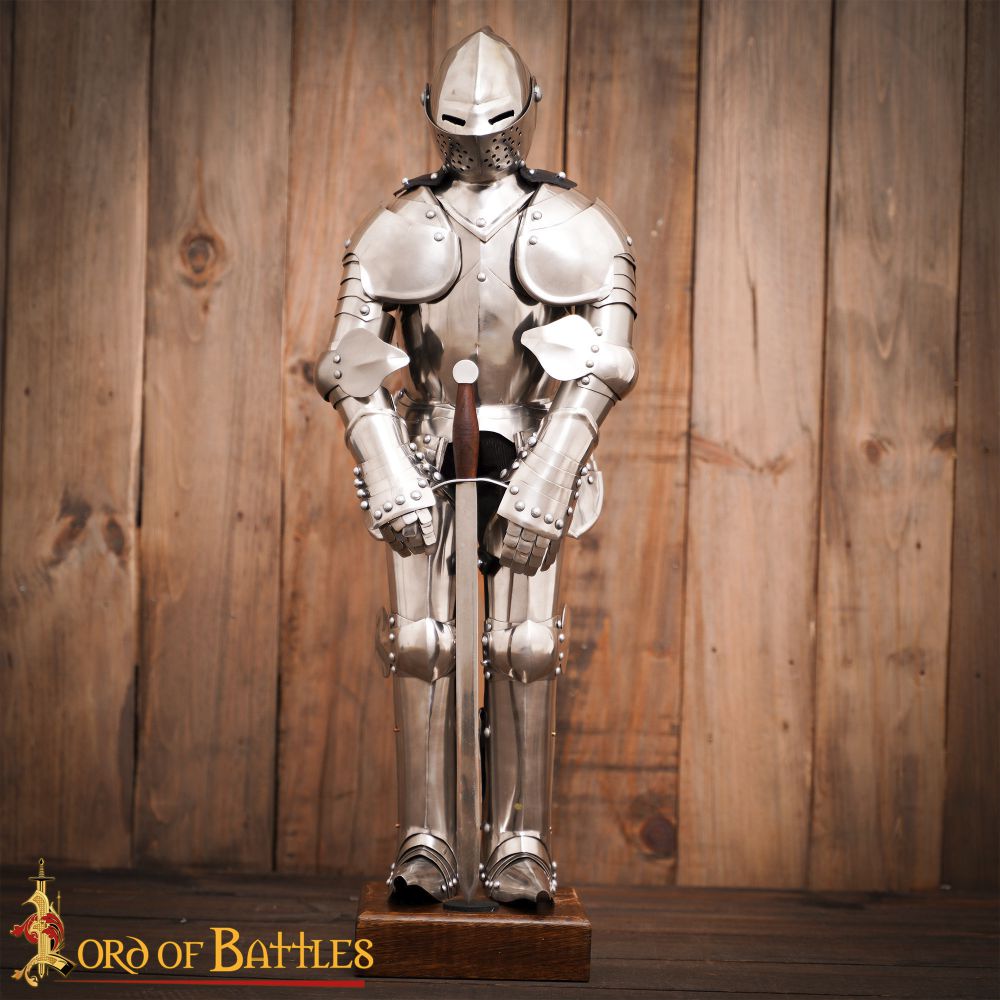The image showcases a full suit of knight's armor, meticulously detailed and presented on a dark brown wooden pedestal, situated in a rustic room with wood-paneled walls. The gleaming, chrome silver armor covers the entire body from head to toe, including the helmet, which features two rectangular eye slits and a perforated mouthpiece that can lift to reveal the face. The arms, chest, shoulders, legs, feet, and even the fingers are protected by this intricate metal casing. At the center, the knight holds a large, silver sword with a brown handle, its tip resting against the pedestal. A prominent inscription at the bottom left-hand corner of the image reads "Lord of Battles." The natural wood backdrop enhances the prominence of the knight, highlighting the craftsmanship and historical essence of the armor.